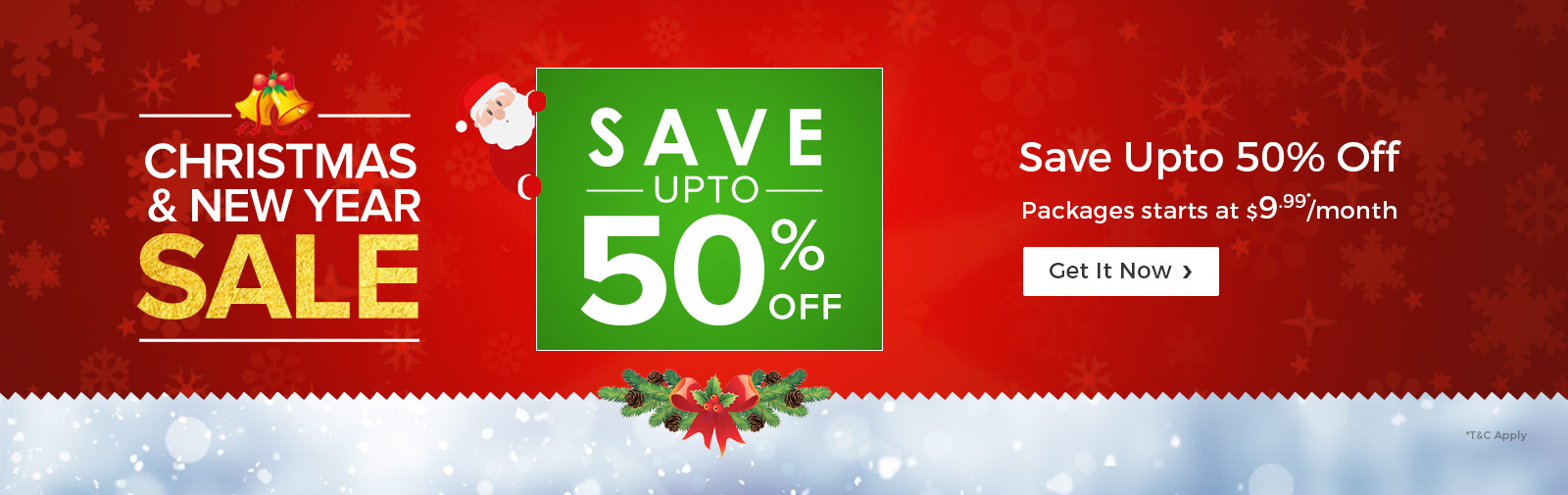This festive website banner, designed for the holiday season, exudes warmth and cheer. The upper three-fourths of the image is a vibrant red, adorned with delicate snowflakes and star symbols. This section ends in a playful zigzag pattern reminiscent of the torn edge of wrapping paper.

On the left side, yellow bells, vivid red berries, and swirling ribbons frame the text "Christmas and New Year's Sale," enhancing the festive spirit. A green square occupies the center of the banner, detailed with white text proclaiming "Save up to 50% off." From behind this square, Santa Claus jovially peeks out from the upper left corner. Below the text, a charming green wreath decorated with brown pinecones and a bright red bow adds a touch of traditional holiday decor.

The top right corner hosts a promotional message repeating "Save up to 50% off," followed by an enticing offer, "Packages starting at $9.99 a month," and a prominent "Get Now" button for immediate action.

The bottom one-fourth of the image transitions into a serene sky blue, speckled with white circles and flakes, artfully mimicking falling snowflakes to complete this enchanting holiday scene.